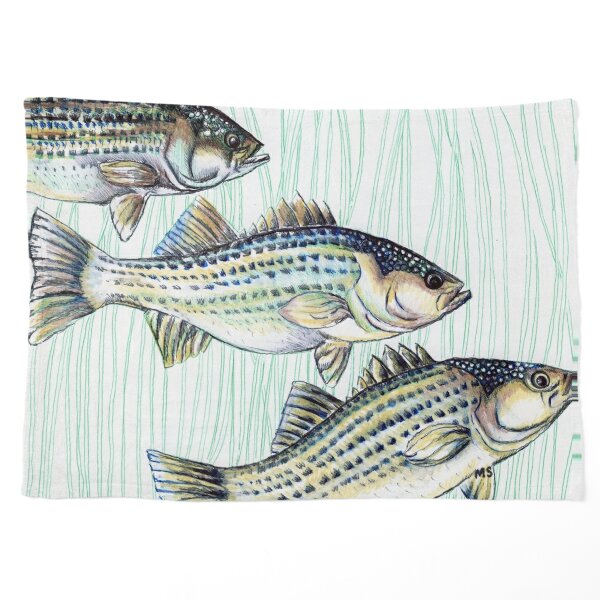This image depicts a textile artwork, likely on fabric, possibly a pillowcase, featuring three colorful fish. The fish appear to be swimming through a green, water-like background, crafted with green lines and possibly designed to simulate aquatic movement. 

The upper left fish faces forward with visible fins but a hidden tail. In the middle, the second fish has blue on its upper body with hints of green and tan, its fins and tail fully visible. The third fish, located at the bottom middle and tilting upwards, displays similar hues of green, tan, and blue, with notable black and white scales on its face and body.

Common among all three fish are their black and white spots and gills. The background, predominantly green, suggests an underwater setting. Detailed observations reveal the initials "MS" at the bottom, implying the artist's signature. The artwork showcases a broad palette, featuring blues, blacks, yellows, greens, and whites, effectively bringing the fish to life as they appear to swim toward an opening in the scene.